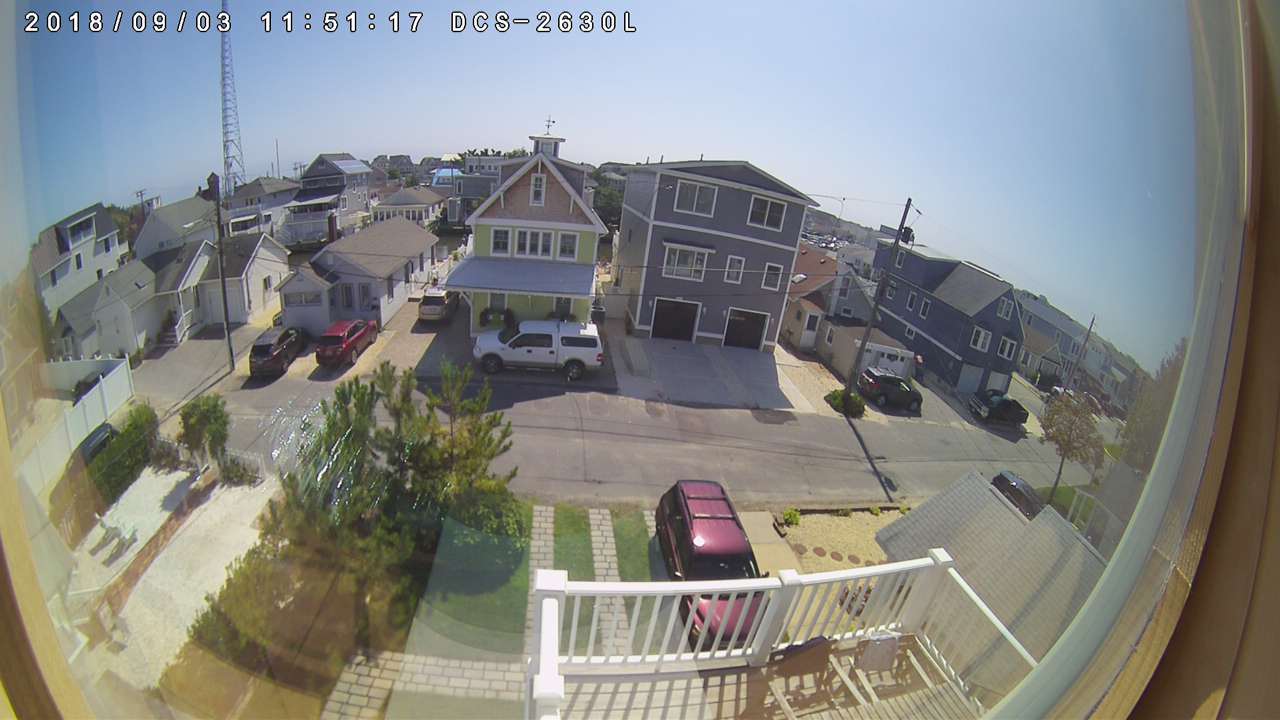This image, captured from a security camera located on the upper floor of a house, possibly the second or third floor, dates back to March 9, 2018, at approximately 11:51 AM, as indicated by the timestamp "2018-09-03" and "11:51:17" in white text at the top left corner. The camera model, DCS-2630L, is also noted. The scene showcases a bright, clear day with a vivid blue sky, devoid of clouds. The view encompasses various residential buildings, houses, and complexes arranged around a main street running down the center of the image. On the right side, a white balcony, complete with a few chairs, is visible. Below the balcony, a red van is parked in the driveway. In the front yard, there are two distinct brick paths where vehicle tires go, bordered by a lawn and a fence. To the left side of the image, a tall electrical or cellphone tower can be seen in the distance, alongside other houses interspersed with trees. A white car is parked horizontally across the street, adding to the suburban feel of the neighborhood captured in this wide-angled, slightly fisheye distorted security camera snapshot.